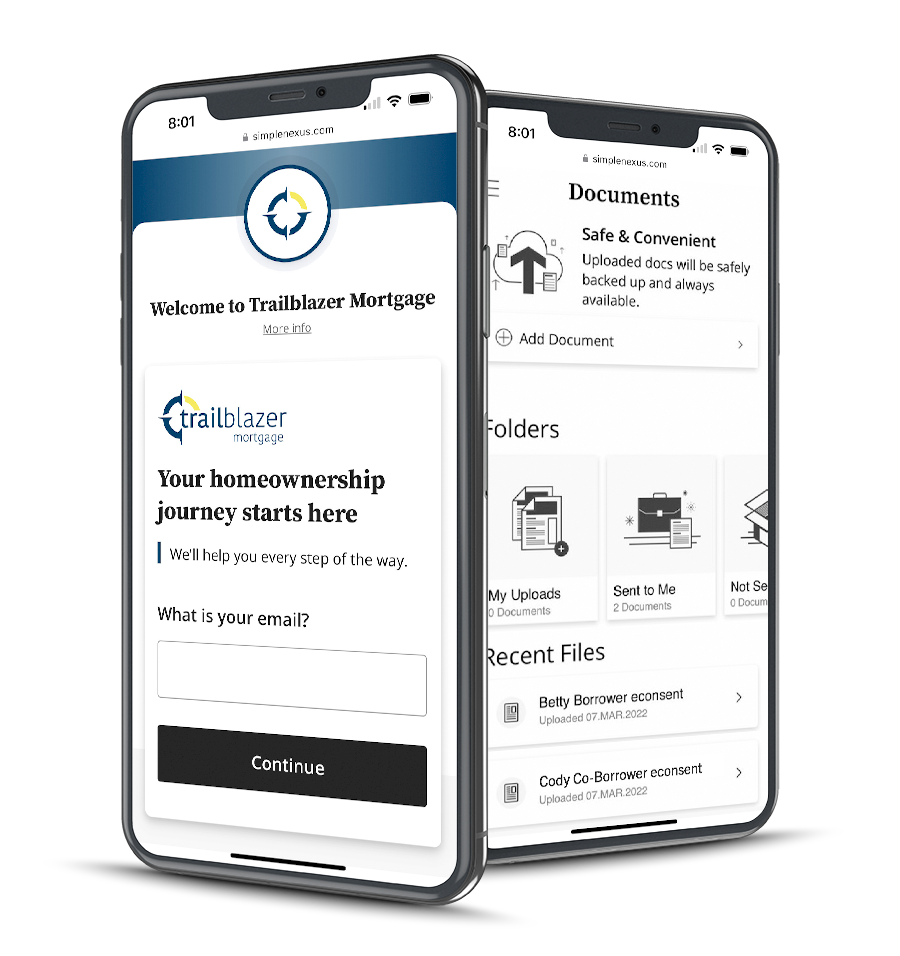The image displays two smartphones, reminiscent of those seen in cell phone advertisements or refurbished phone listings. Both devices share the same style and appear to be in dark colors, either black or dark gray. The phone on the left is tilted towards the left and positioned closer to the viewer, while the phone on the right is tilted towards the right and set slightly further back.

The phones show identical times and similar notifications, including indicators for cell phone service, Wi-Fi, and battery status. The background of the phone on the right is completely white, whereas the phone on the left features an ombre effect at the top, transitioning to a lighter blue color in the center.

On the left phone, a singular company logo is visible. In contrast, the right phone displays a variety of basic, clip art-style icons commonly found in a phone’s settings menu. The overall presentation and alignment of the devices evoke the aesthetic of commercial product displays, emphasizing their sleek design and functional interface.